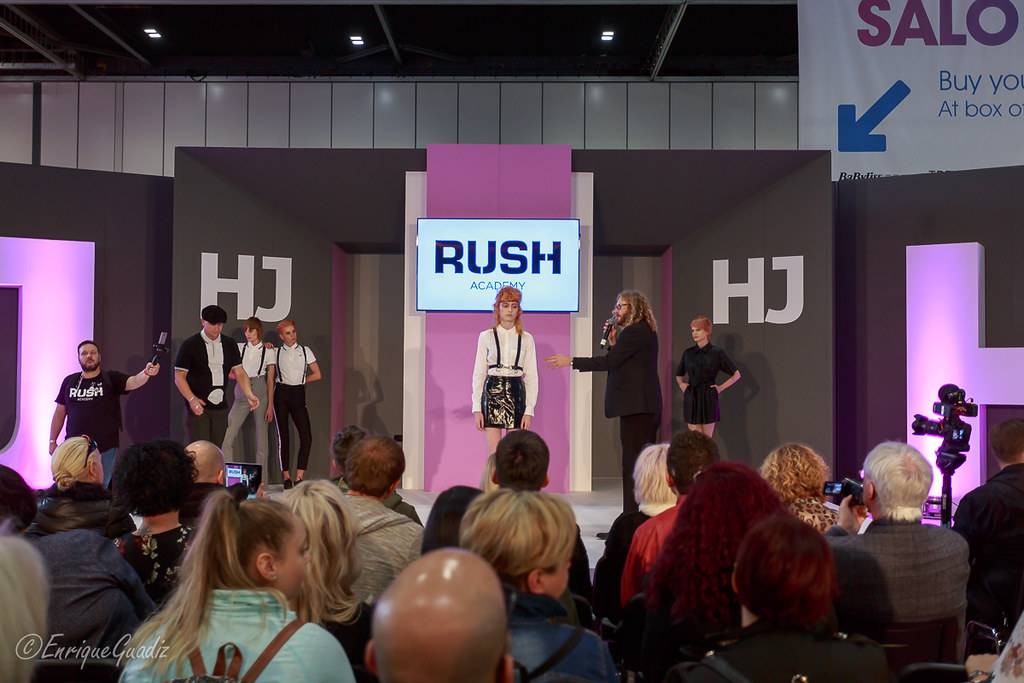In the image, a model, distinctive with her red shoulder-length hair, is walking down a stage lined with people on both sides. She is dressed in a long light-sleeved shirt, a black skirt, and black suspenders, with her hands hanging straight down and her eyes seemingly closed. To her right, a man in a black suit with glasses, a beard, and long curly gray hair, extends one hand toward her while holding a microphone with the other. Behind him stands a woman in a black suit with her hands on her hips against a gray wall. On the left side, there are three men against the gray wall, with another man behind them in a black "Rush" shirt, holding up a microphone. The gathered audience in the foreground includes a bald man reflecting light off his head, a girl with tightly pulled-back blonde hair and a red and light blue collared jacket with a backpack, and a woman with short blonde hair in a blue coat.

A large lit-up screen at the back displays "Rush Academy," with gray walls on either side marked with 'H' and 'J.' The upper right corner features part of a white banner with a blue arrow pointing downward, spelling out "S-A-L-O" in purple letters beside "B-Y-O" and "Atbox O" below. The setting suggests a conference or presentation, with various people holding cameras to document the event.